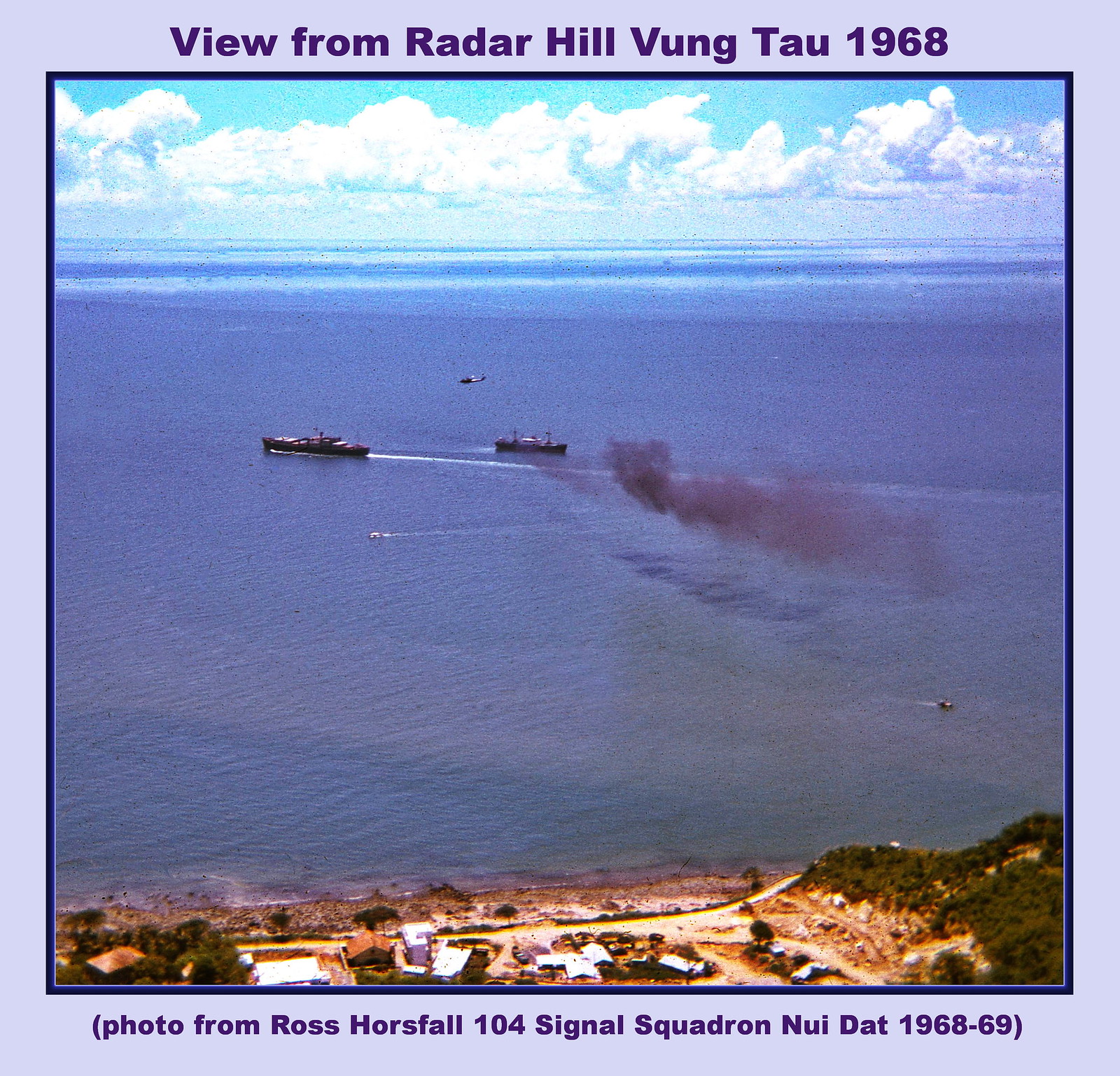The square postcard titled "View from Raider Hill, Vung Tau, 1968" captures a sweeping vista focused mainly on a waterway or ocean with a light purple border framing the photograph. At the bottom, it notes: "Photo from Ross Horsefall, 104 Signal Squadron, Newell Det, 1968-1969." Dominating the scene are two larger boats, one trailing smoke, alongside a few smaller boats dispersed across the water. Above, a helicopter hovers in clear blue skies dotted with white clouds. The bottom section reveals a shoreline featuring dilapidated buildings, dirt roads, and patches of greenery, suggesting a war-torn landscape consistent with Vietnam circa 1968.